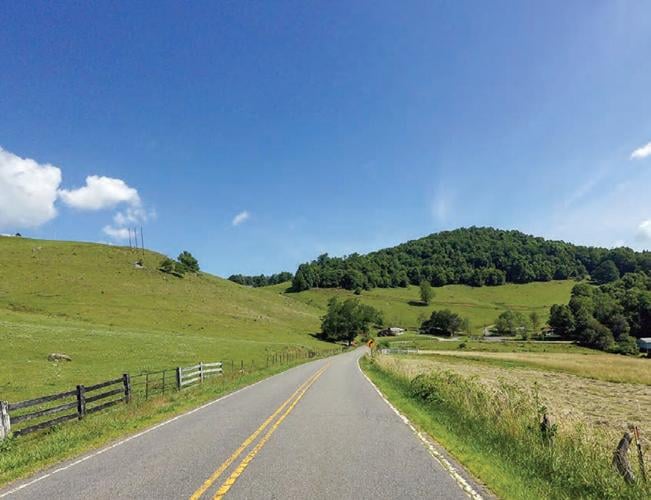A picturesque photograph captures a single-lane road meandering through verdant rolling hills, flanked by differing landscapes on each side. The road, paved with black asphalt and marked by double solid yellow lines at its center and white lines along the edges, stretches from the foreground into the distance, gently curving to the right as indicated by a yellow road sign ahead. To the left of the road, an old wooden fence borders lush grassy hills, which gradually rise into a dense tree-covered slope that meets a partly cloudy, vivid blue sky. On the right, the land is flatter, featuring open green fields and a wire fence, transitioning into a hill adorned with dark green trees. Three poles stand out against the backdrop, contributing to the serene countryside vista. In the distant background, a few scattered buildings nestle among the trees, completing this idyllic scene bathed in midday sunlight.